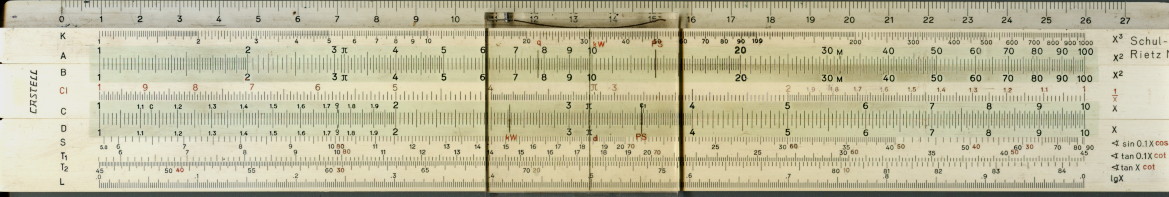A close-up photograph showcases a white plastic scale ruler, prominently featuring various measurement scales. At the top, there is a centimeter scale clearly printed, and below it are two sliding black lines designed to convert centimeters to inches and other metric measurement systems seamlessly. The brand name "Castel" is visibly printed on the left side of the ruler in bold text. On the right side, additional black text details names of different measuring systems. The image is tightly cropped, focusing exclusively on the elongated, thin ruler, with no other objects visible in the frame.